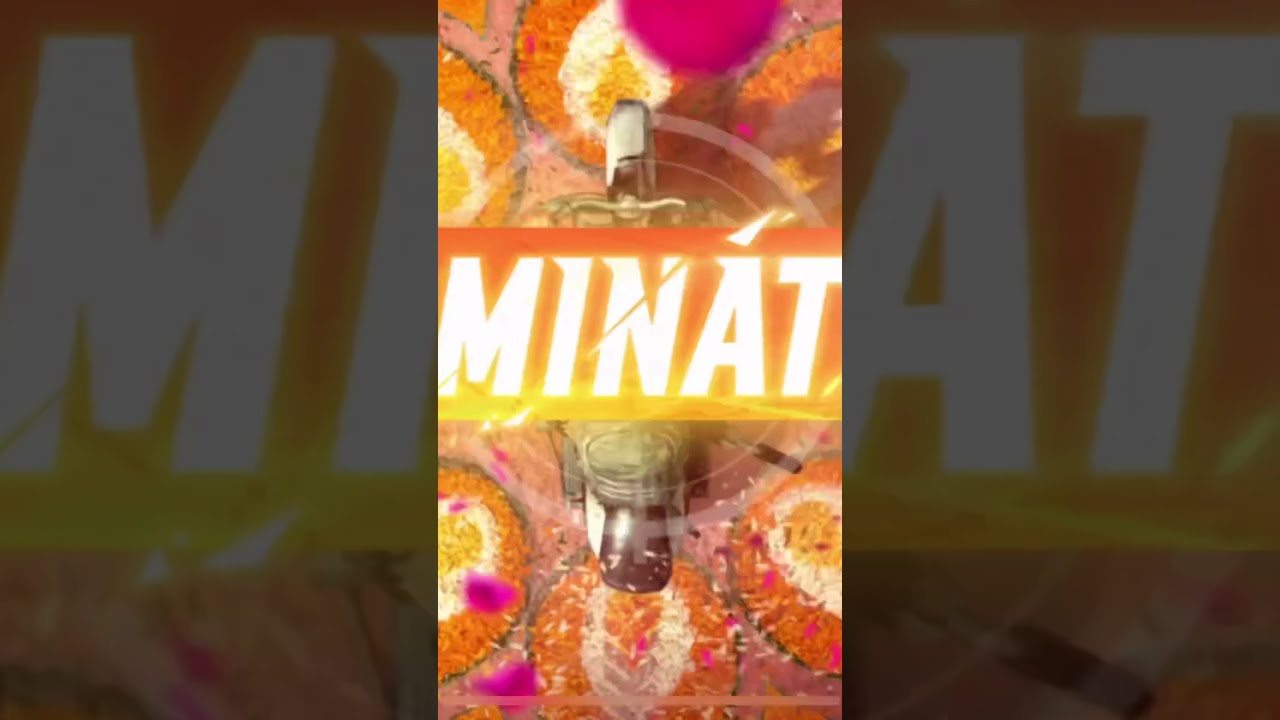This vertical poster is divided into three sections from top to bottom, with the left and right thirds having a darker palette compared to the bright, vibrant center section. On the left side, the dark area is adorned with the capital letters "MI" in a mix of yellow, white, cream, and hints of pink. The right section mirrors this, showcasing the capital letters "AT" in the same color scheme. 

The central third of the poster bursts with vivid colors—bright pinks, yellows, whites, oranges, and purples—resembling a collage made from various colored seeds. An orange and yellow banner spans horizontally across the middle of this section, containing large white capital letters spelling "M-I-N-A-T." 

Beneath the banner, there appears to be a top-down view of a motorcycle, with its handlebars at the top of the banner and the rear seat and tire at the bottom. The detailed orange circles surrounding the motorcycle resemble flames or intricate designs on the ground. Shadows to the right of the motorcycle add depth, further suggesting its presence.